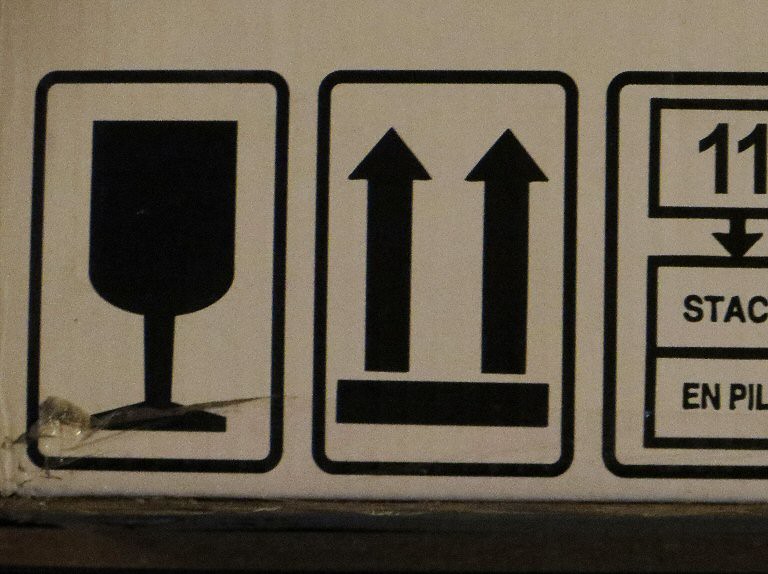This photograph showcases a white and black sign adorned with various symbols, positioned on a gray shelf. The sign is divided into three sections, each framed by black rectangles with rounded corners. On the far left, there is a depiction of a stylized black cup, complete with a stem, base, and bowl. The center section features two long, upward-pointing arrows side by side, underlined by a horizontal black bar. The rightmost section of the sign is partially cut off but displays the number "11" prominently, followed by the letters "S-T-A-C." Below this, fragmentary letters "E-N-P-I-L" can be discerned.